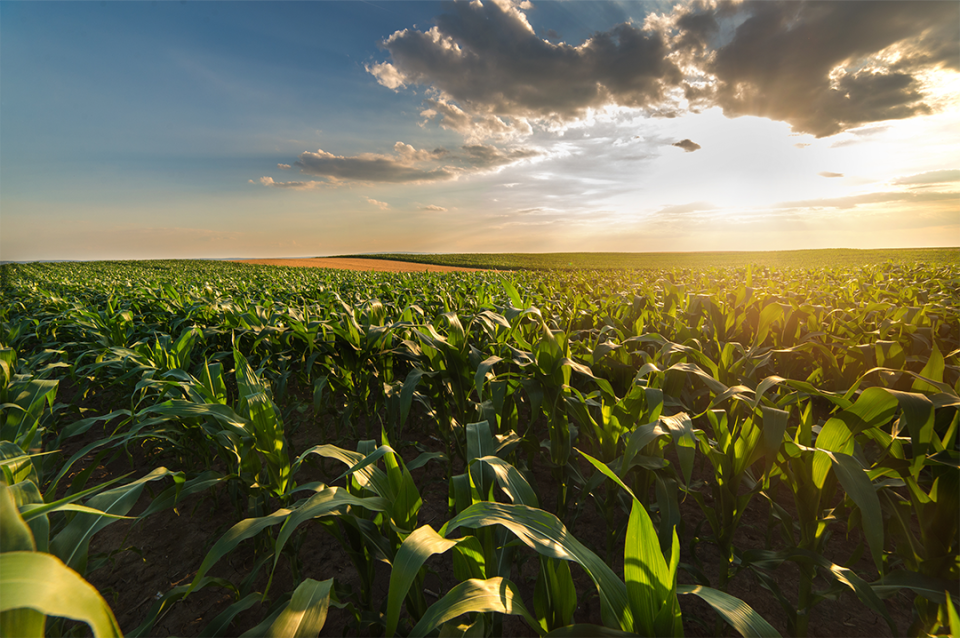In this stunning outdoor image taken in a Midwest setting during a beautiful mid-afternoon, the sun is prominently close to sundown, casting a warm, golden hue across the scene. The sky is a brilliant blue with scattered clouds, creating a picturesque backdrop. Dominating the image is an expansive, meticulously cultivated field filled with thousands upon thousands of uniformly green-leaved crops, reminiscent of corn but lacking the central yellow stalk, suggesting an early growth stage. This vast field stretches endlessly towards the horizon. The field is slightly inclined on the left side, adding a gentle curve to the landscape. Dividing the fields is a tan-colored section, possibly a fallow area left to regenerate or intended for future cultivation. This section contrasts with the vibrant green of the crops, and the sunlight highlights the long leaves, emphasizing the meticulous agricultural maintenance that characterizes the scene.